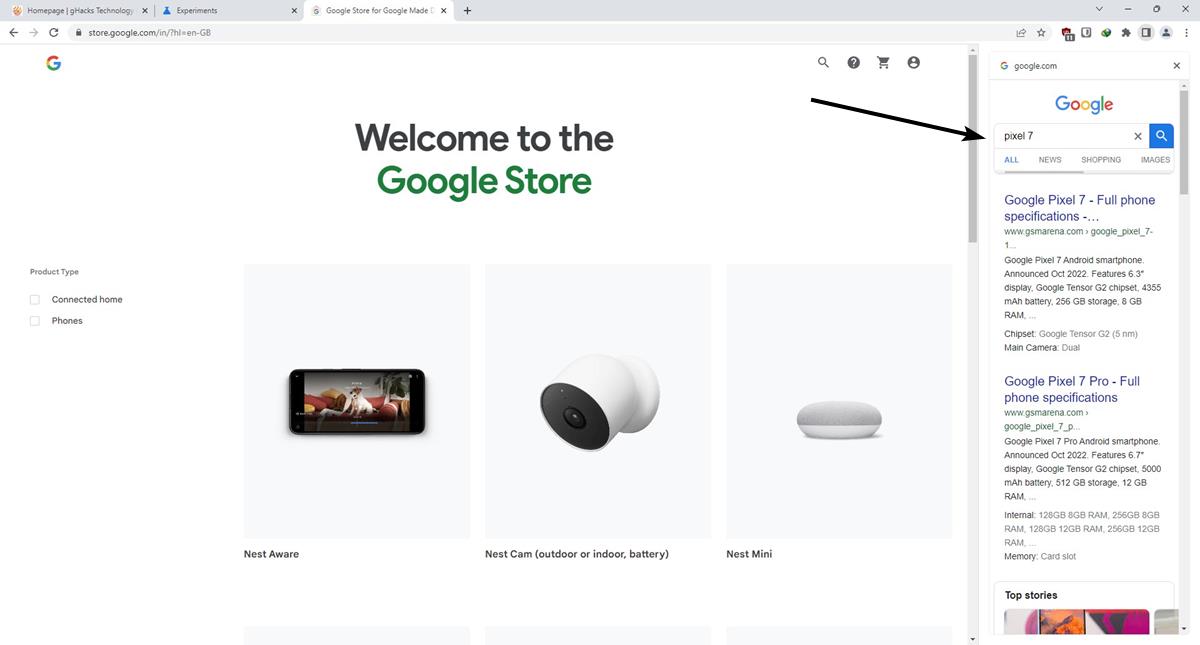This is a detailed screenshot of the Google Store interface being accessed through a web browser. The browser window is relatively small, making finer details hard to decipher. Despite this, the screen maintains a clean, predominantly white design. 

On the right-hand side, there's a panel displaying various products available in the store, complete with detailed clickable areas. The main section prominently features a welcome message, "Welcome to the Google Store," with the words "Google Store" highlighted in green. The Google logo is positioned in the upper left corner, while the upper right corner contains simplified menu icons for search, shopping cart, and profile information.

An overlaid black arrow points towards one of the search results, which appears to be for the "Pixel 7." This right-hand column seems to be filtering search results within the Google Store.

Centered in the main area is an image of a smartphone laid on its side, accompanied by a picture of a Nest Camera and another device, possibly a Nest Mini, which resembles a small voice assistant. The product category "Connected Home" headings these items, with images illustrating the three types of products. A vertical scrollbar on the right side of the panel suggests additional items are viewable upon scrolling.